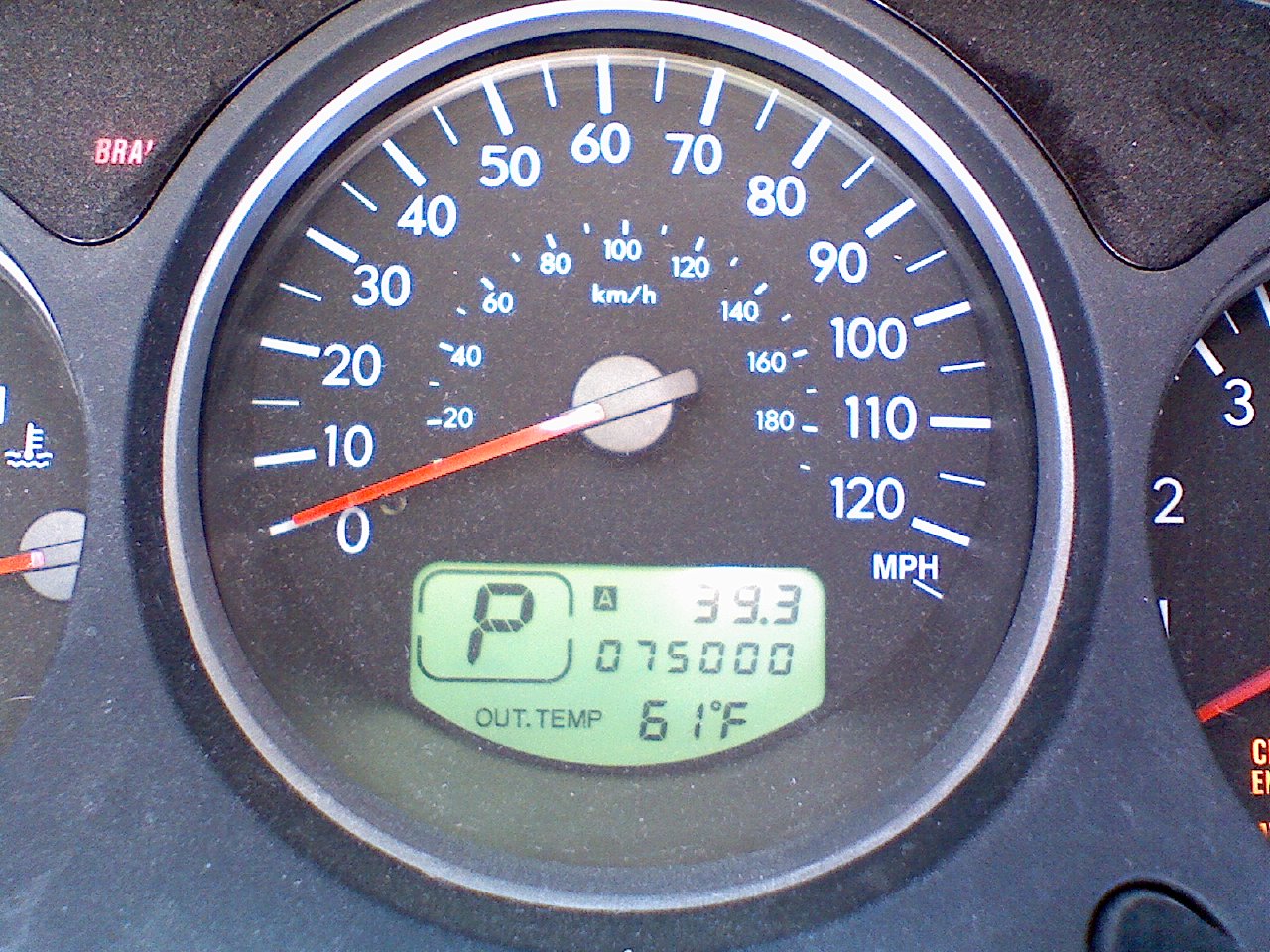This photograph is a detailed close-up of the speedometer on a car's dashboard. The central speed gauge, a large black circular dial with a gray border, prominently displays white numbers ranging from 0 to 120 miles per hour in 10 mph increments. An inner band shows kilometers per hour from 20 to 180 kph. A long narrow orange and black indicator rod points to zero. Below the gauge, a green LED screen displays several readouts: "P" indicating the gear, "39.3" for trip mileage, "075000" for the total mileage, and "Out Temp 61°F" for the outside temperature. The image also captures the edges of two other meter displays on either side, with the left showing part of a brake light, and the right showing a gauge with the numbers 1, 2, and 3.